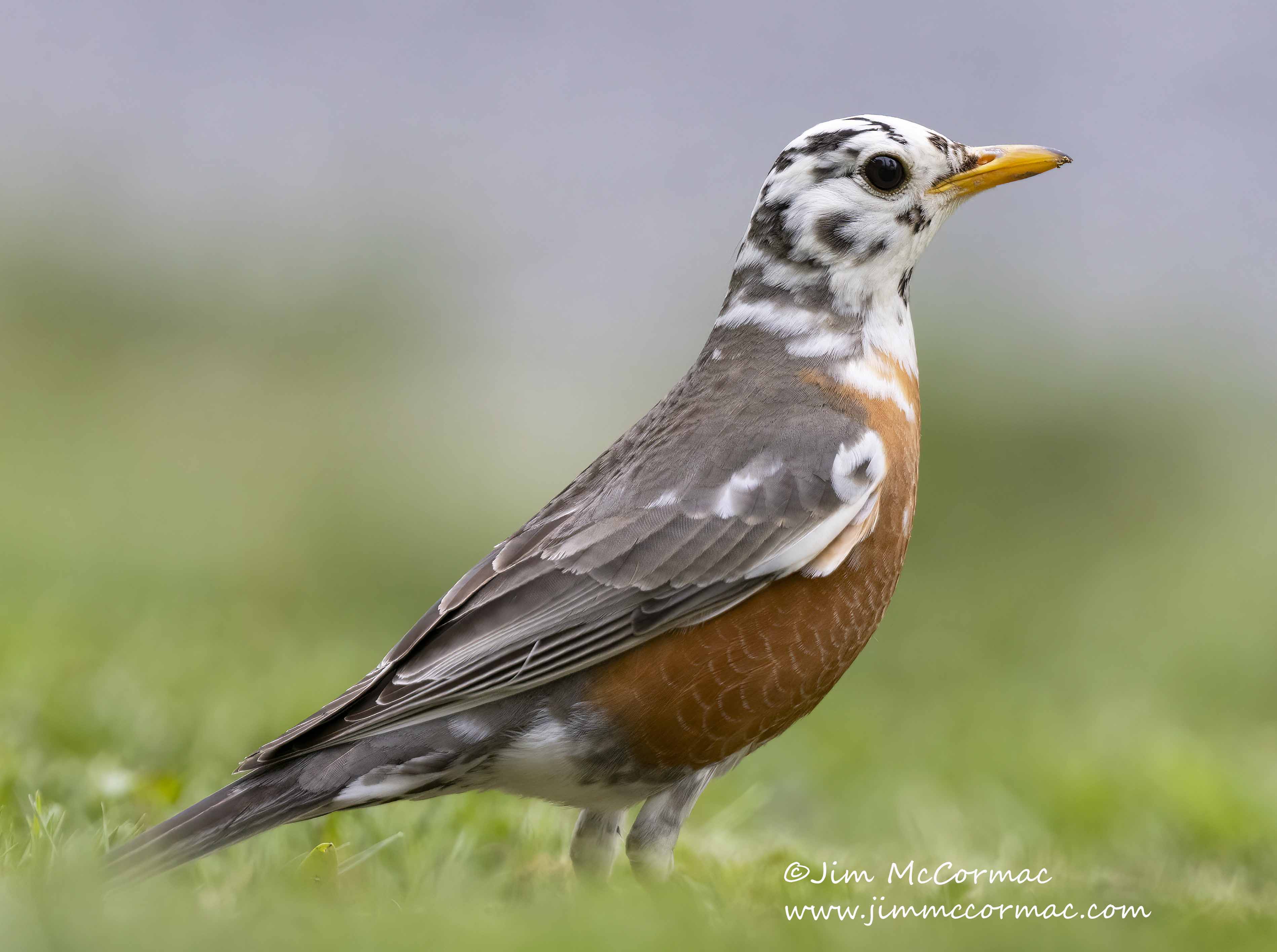This detailed close-up photograph, taken by Jim McCormick, captures the stunning side profile of a uniquely colored bird with remarkable clarity. The bird features a striking white head adorned with black markings that resemble swirls, not stripes, accentuated by a black eye and a vivid yellow beak. The intricate plumage includes primarily black wings speckled with white spots, a reddish belly, and a white underside with black spots on its legs. The background, skillfully blurred, suggests a grassy field with hints of gray, allowing the bird to stand out sharply in the foreground. The bird appears to be no larger than a sparrow, possibly a type of grackle, distinguished by its naturalistic and realistic presence. At the bottom of the photo, a watermark crediting Jim McCormick directs viewers to his website, www.jimmccormick.com, for more information.